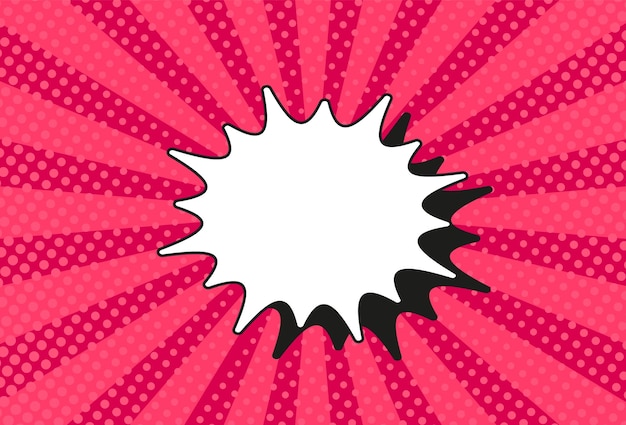This is a vivid cartoon-style illustration featuring a central, large white splatter, reminiscent of a glass of milk or putty thrown down that has splattered. The splatter has a pronounced shadow extending toward the bottom right, adding a sense of depth. This center splatter could evoke comic book sound effects like "BAM" or "POW," hinting at its dynamic nature. The background is composed of vibrant pink and dark red rays radiating outwards like a starburst, with a pattern of light pink polka dots evenly spread across. The whole scene exudes a colorful, psychedelic energy akin to classic comic book action panels.